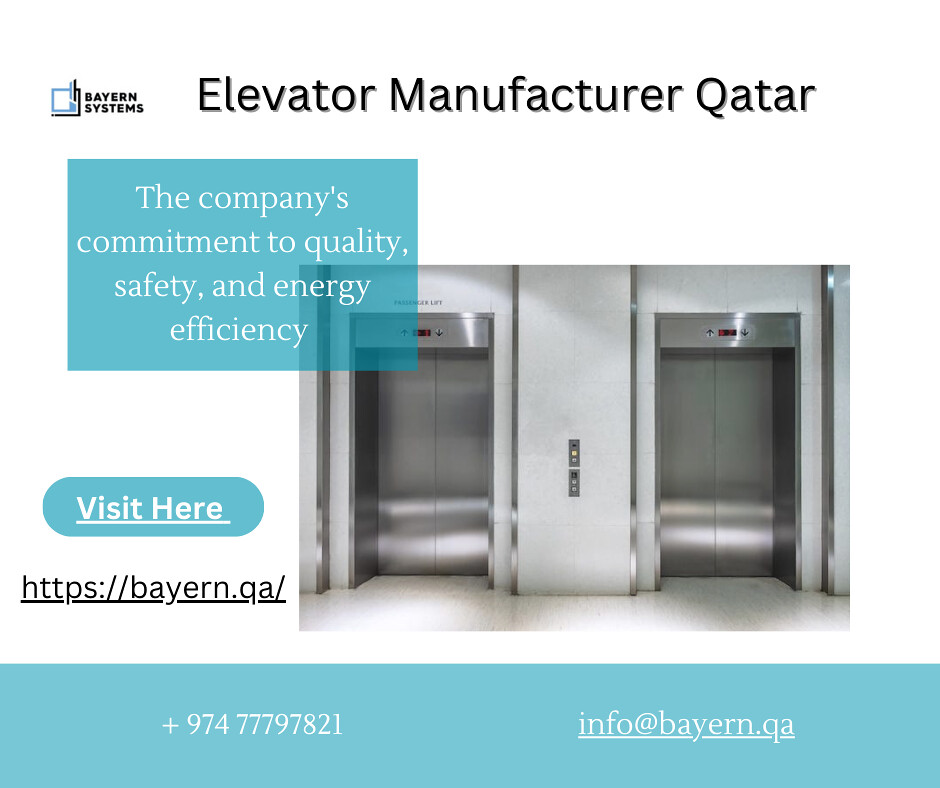The image is an advertisement for Elevator Manufacturer Qatar, prominently displayed in black text atop a white background. Adjacent to this, on the upper left, is the Bayern Systems logo, featuring a small white and blue square. Beneath these titles is a blue box containing white text that reads, "The company's commitment to quality, safety, and energy efficiency." Below this, a small blue circle with white text invites viewers to "Visit here." 

At the center of the image is a photograph of two steel grey elevator doors situated within a white wall, flanked by buttons. The floors are also white. Near the photograph, the website "https://bayern.qa" is noted. The bottom of the image includes a light blue rectangle with white text displaying the company's contact information: phone number "+974-777-97821" and the email address "info@bayern.qa".